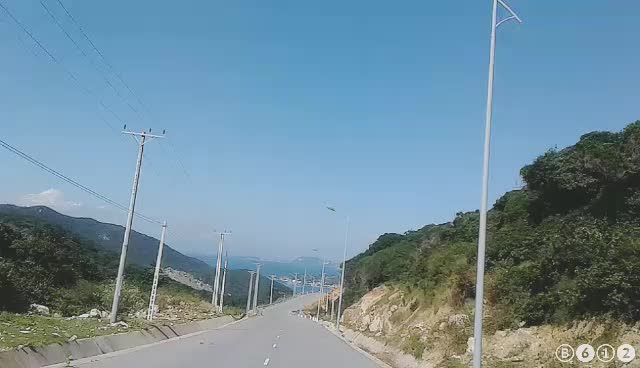The photograph, likely captured by a dash cam, depicts a two-lane concrete road winding through a mountainous region. This road, characterized by its white surface and distinct white markers, snakes through valleys, offering a scenic route through the mountain pass. Power lines on T-shaped poles line both sides of the road, providing electrical connections and featuring streetlights on the right-hand side. The left side of the image displays rocky, green hills that ascend towards the mountain peaks, with a clearer view of mountains further back, showing a gradient from green to a bluish tone in the distance. The sky, predominantly blue, transitions from a hazy white near the horizon to a deeper blue at the top, dotted with a few white clouds. The right side mirrors the left with rocky hills and lush vegetation, interspersed with numerous trees and tall streetlights. The photograph is grainy and of low quality, and in the bottom right corner, four symbols are visible: B, 6, 1, 2, arranged in a manner suggesting the label "B612". The overall scene indicates a bright summer or tropical day in a very mountainous and green area.